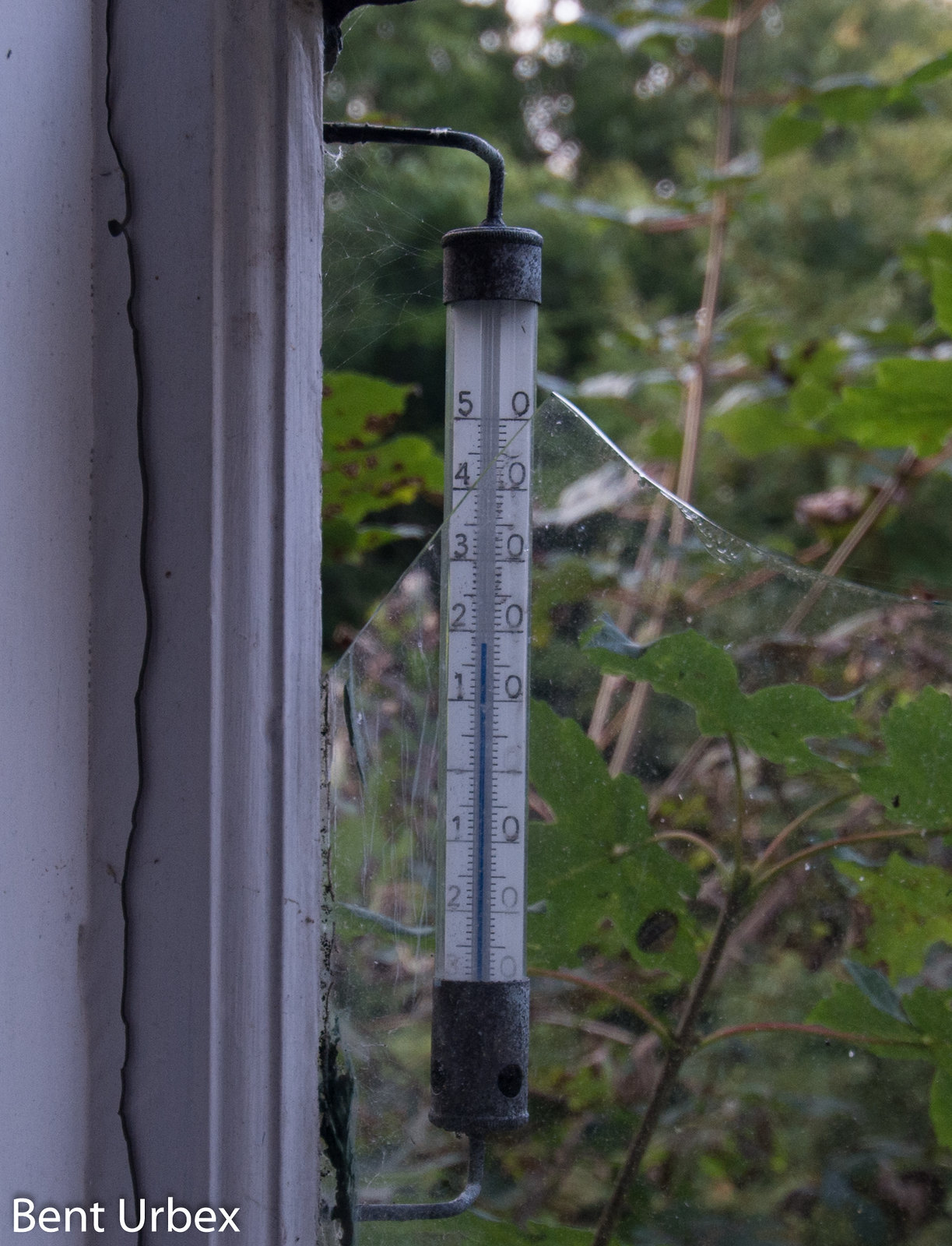In this evocative photograph taken through an old, weathered window, the details of decay and nature's tenacity are captured vividly. The window frame, encrusted with peeling white paint, surrounds smudged and grimy glass marred by water streaks and broken shards, suggesting years of neglect. Just beyond the fractured pane, affixed to the exterior wall, is an intriguing, unusual temperature reader that resembles a simplistic rain gauge marked with the numbers 1 through 5. This device, though stark and functional, stands out against the backdrop of ruination. Encroaching spider webs cling to the top of the thermostat, adding to the sense of abandonment. The outside world teems with verdant life, as trees, shrubs, and dense foliage form a lush, green tapestry under a summery sky. This striking contrast between the thriving nature and the dilapidated man-made structure creates a compelling scene of serene decay and quiet resilience.